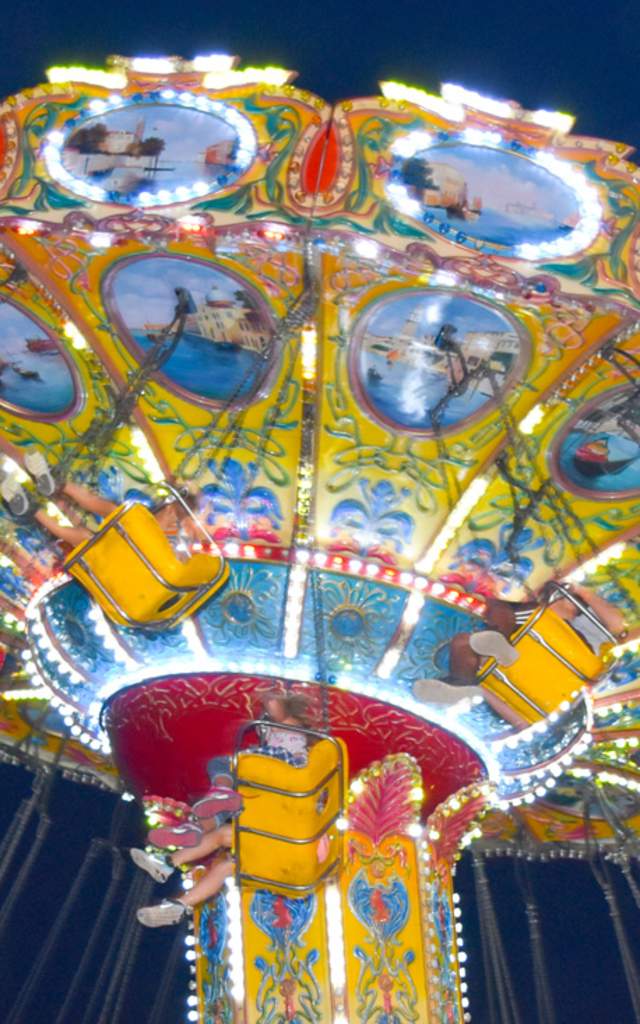This photograph captures the vibrant scene of a carnival ride taken near dusk, accentuated by an array of colorful lights piercing through the dimming sky. The image is looking up at a towering swing ride, approximately 20 feet tall, with swings lifting and revolving around the towering structure. Each swing, painted a bright yellow and attached by chains, gently tilts and lifts the riders as it rotates. Some swings accommodate single riders, while others hold pairs, creating a dynamic aerial dance. The central tower of the ride stands out with its vivid yellow hue complemented by blue and red highlights, adorned with intricate, colorful pictures and scenes on every available space. The base of the ride features a striking yellow with a red circular design. The whole scene, with lights sparkling and multiple people enjoying the ride, exudes a festive, lively atmosphere.